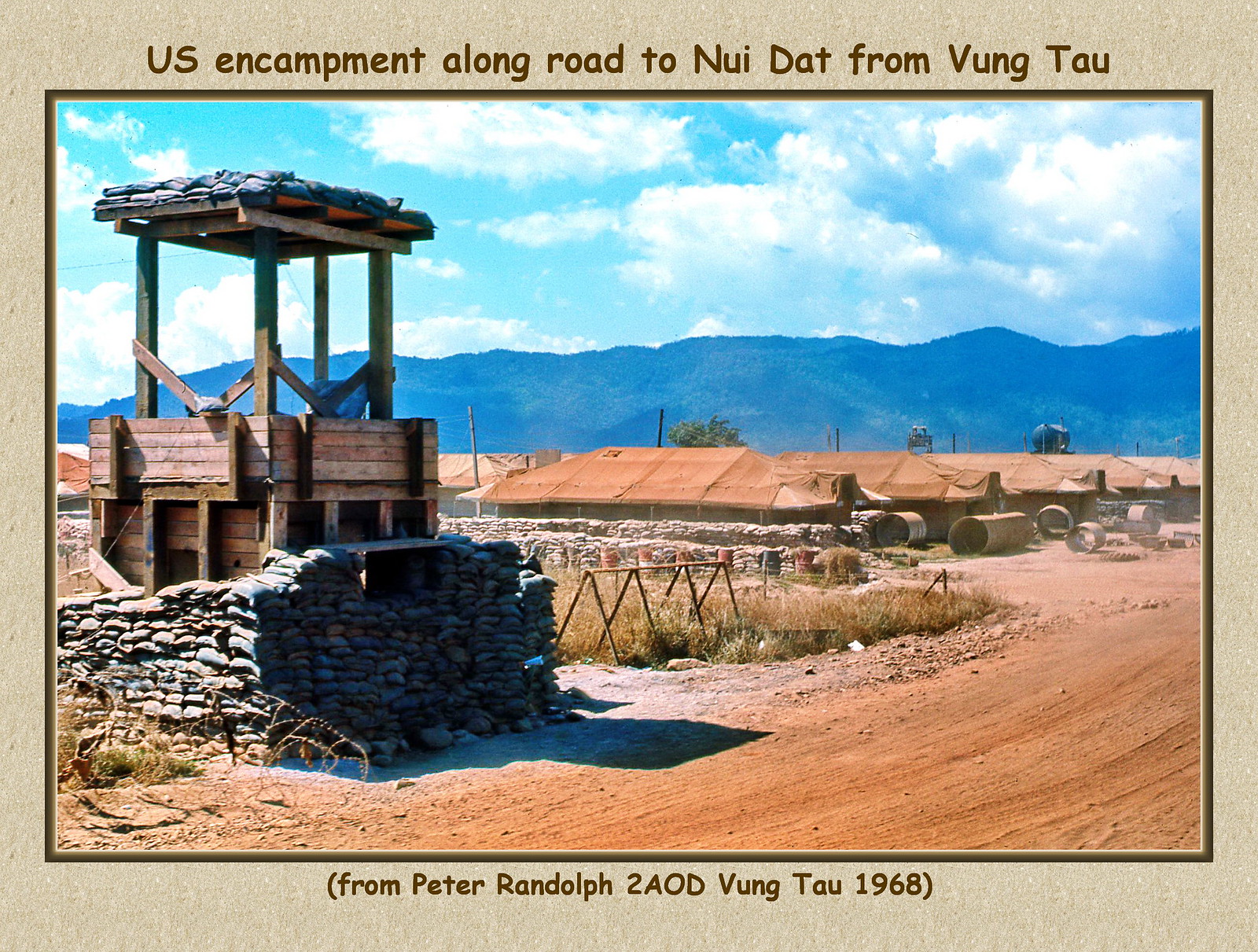This color photograph captures a detailed scene of a historical military encampment. Dominating the left side of the image is what appears to be an old water well, fortified by stacks of sandbags. Above it, a wooden sentry tower, also surrounded by sandbags, stands watch. The surrounding area transitions into a grassy patch leading to a collection of brown tents with additional sandbags piled along their edges. In front of these tents, large circular culverts are positioned. The lower right corner reveals a dirt road that winds through the scene. Beyond the immediate encampment, a striking blue mountain range undulates across the background under a blue sky adorned with scattered white clouds. The image is framed by a brown border, with the top labeled in brown text, "US encampment along road to Nui Dat from Lung Thao," and at the bottom, "From Peter Randolph to AOD Lung Thao 1968" in parentheses.